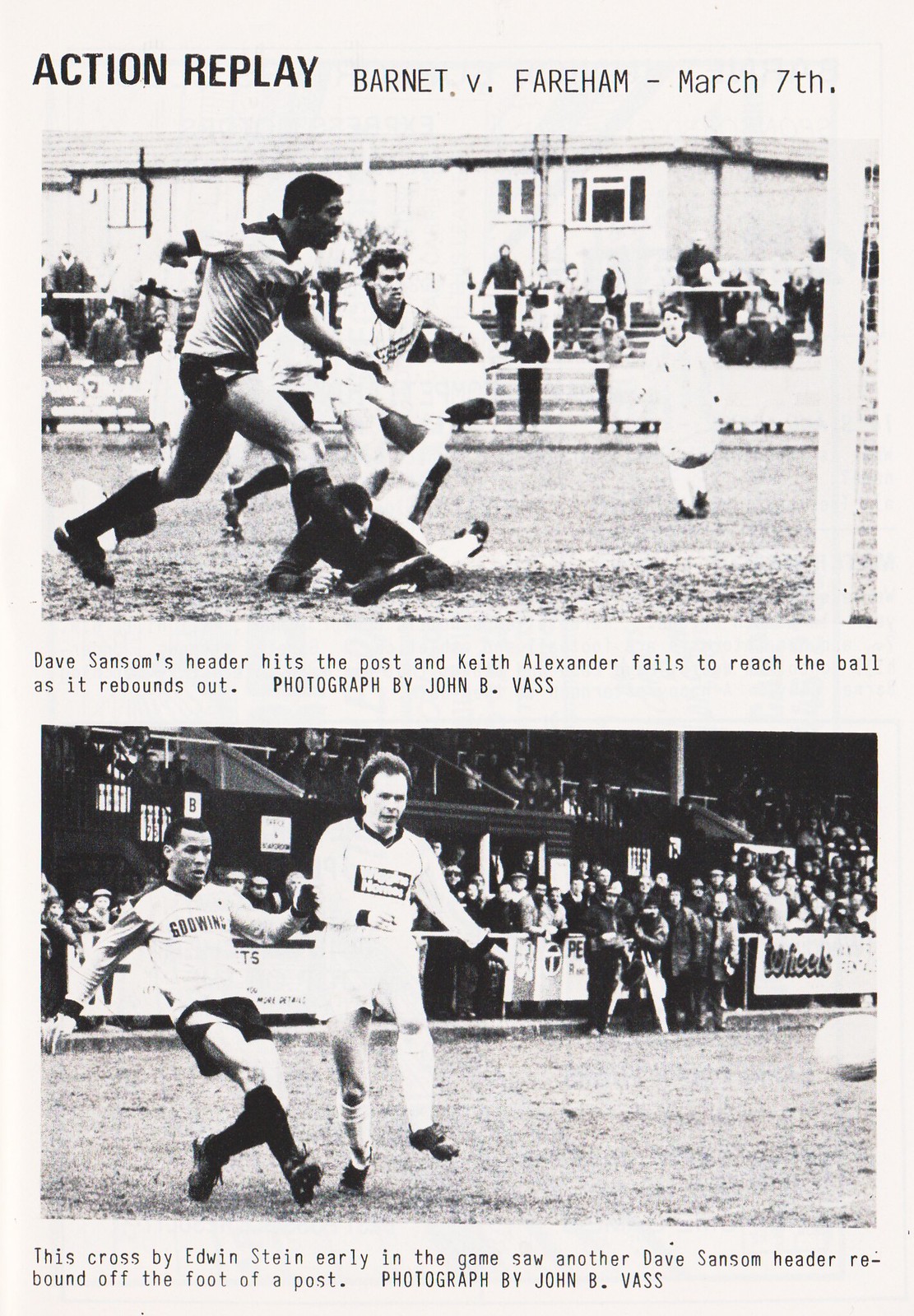The image is a black and white interior page from a sporting magazine, featuring two distinct sections analyzing a soccer match between Burnett and Fairham on March 7th. The top half captures the intense moment of a goalie diving for the ball while a soccer player attempts a header. The accompanying caption reads, "Dave Sampson's header hits the post and Keith Alexander fails to reach the ball as it rebounds out," with the photo credited to John B. Vass. In the background, spectators can be seen watching the action unfold. The bottom half of the page showcases another dynamic soccer moment: two players running towards the ball. The accompanying text states, "This cross by Edwin Stein early in the game saw another Dave Sampson header rebound off the foot of the post," and is also photographed by John B. Vass. In both images, the assembled crowd in the stands adds to the atmosphere of the sporting event.